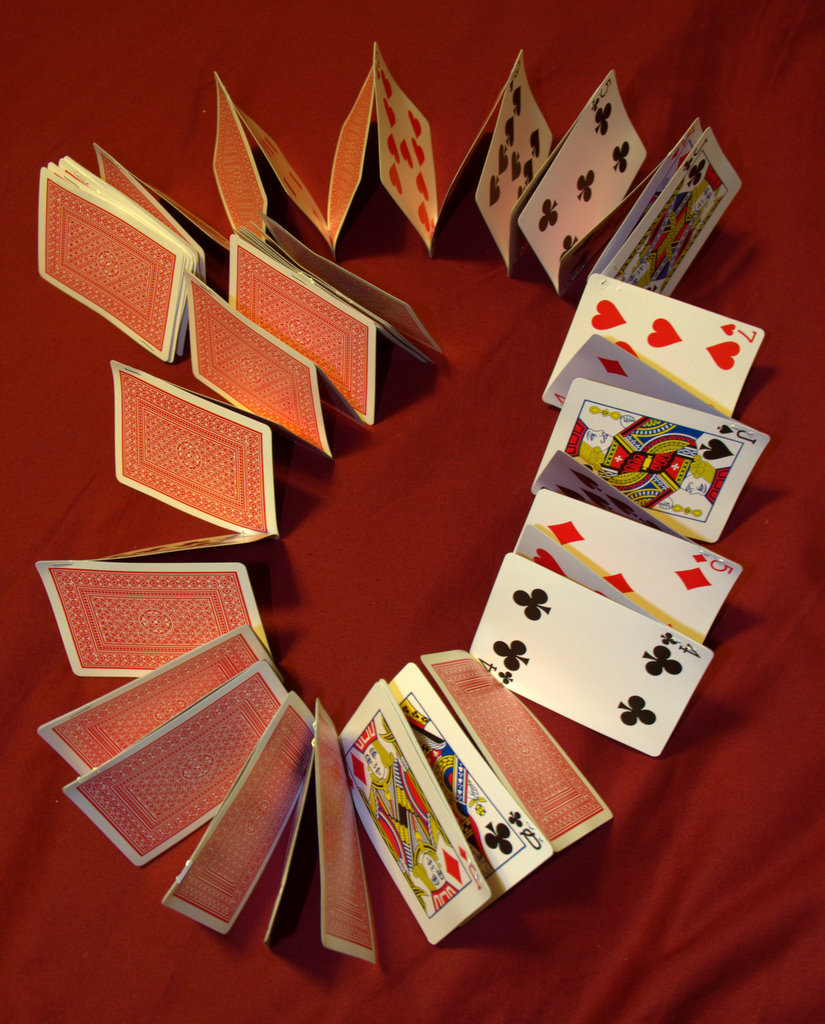This overhead photograph captures a cranberry red tablecloth, slightly wrinkled at the bottom right corner, setting a rich backdrop for an intricate arrangement of playing cards. Formed in an oval or circular shape, the cards are meticulously balanced on their long edges, supporting each other in a delicate display of equilibrium. The visible face cards within the oval include: the King of Diamonds, the Queen of Clubs, the Four of Clubs, the Five of Diamonds, the Jack of Spades, the Seven of Hearts, the King of Clubs, the Five of Clubs, the Nine of Spades, and the Nine of Hearts. On the right side of the arrangement, the face cards are prominently displayed, revealing a variety of suits and values. Conversely, the left side features the backs of the cards, showcasing an intricate red pattern. This artistic composition is not only a testament to balance but also a visually captivating study of color and symmetry.